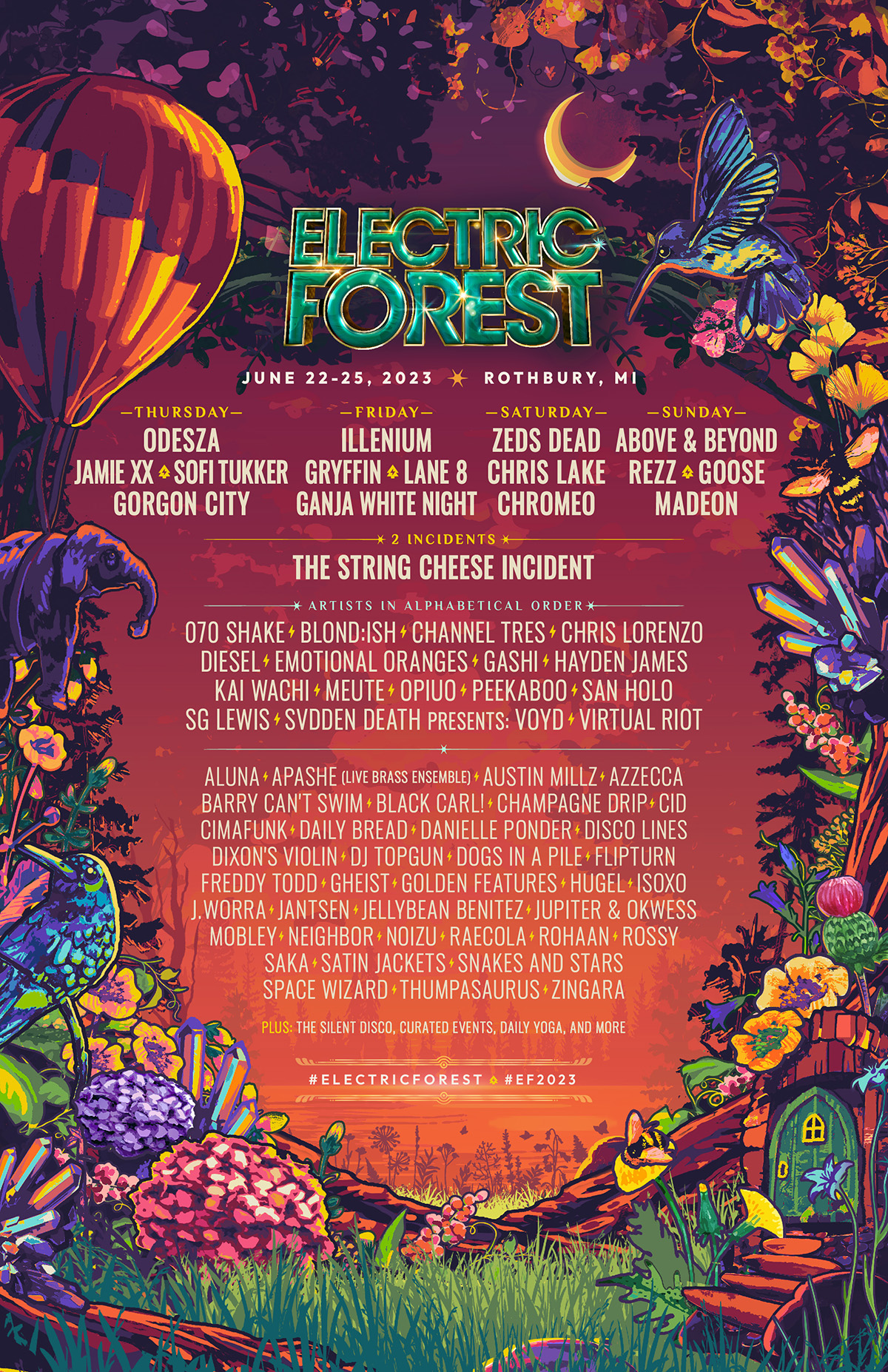This vertical rectangular image serves as an advertisement for the "Electric Forest" concert. At the top, in prominent green text outlined with black and yellow lines, the event name "Electric Forest" is displayed. Just beneath, the dates "June 22nd to 25th, 2023," and the location "Rothbury, MI" are noted.

The central section of the advertisement lists the performance schedule, detailing which artists are performing on each day. The headliner "The String Cheese Incident" is prominently featured among a host of other artists’ names, all written in white text against the vibrant background.

Encircling the central information is a whimsical collection of illustrations, including various shapes, flowers, fantastical figures, birds, butterflies, and balloons. Prominently, a luminous moon shines amidst the enchanting scenery. At the bottom, lush grass provides grounding for the mesmerizing imagery. On the bottom right, there's a quaint, tiny door nestled into a tree, hinting at a magical entryway into the Electric Forest.